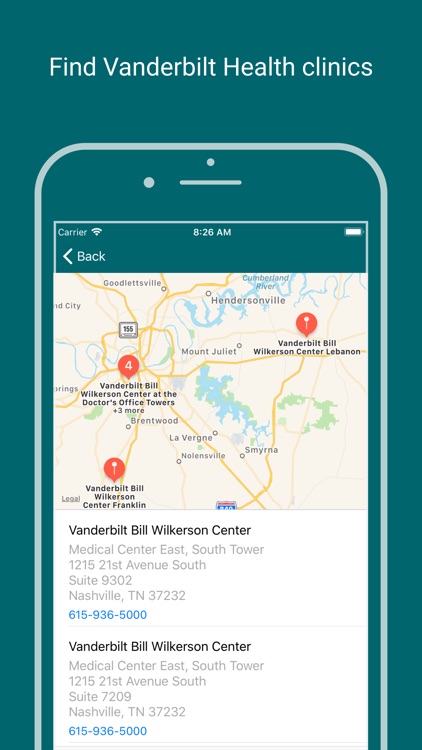The image depicts a mobile application interface designed to help users locate Vanderbilt Health Clinics. The top section prominently displays the heading "Find Vanderbilt Health Clinics," indicating the app's primary function. Below this, a detailed map highlights three specific clinic locations: Vanderbilt Bill Wilkerson Center at the Doctor's Office Towers, Vanderbilt Bill Wilkerson Center in Lebanon, and Vanderbilt Bill Wilkerson Center in Franklin. 

The map also includes other city names like Brentwood, Mount Juliet, Hendersonville, Goodlettsville, and Smyrna, providing a broader context of the metropolitan area, which is revealed to be around Nashville, Tennessee. Further down, the full addresses for two of the clinics are provided, confirming their locations within Nashville.

The entire interface is set against a dark green background, and the image appears to be a mockup rather than an actual screenshot from a mobile device, giving a clear representation of what the phone screen would look like when using the location service feature of the Vanderbilt Health Clinics app.